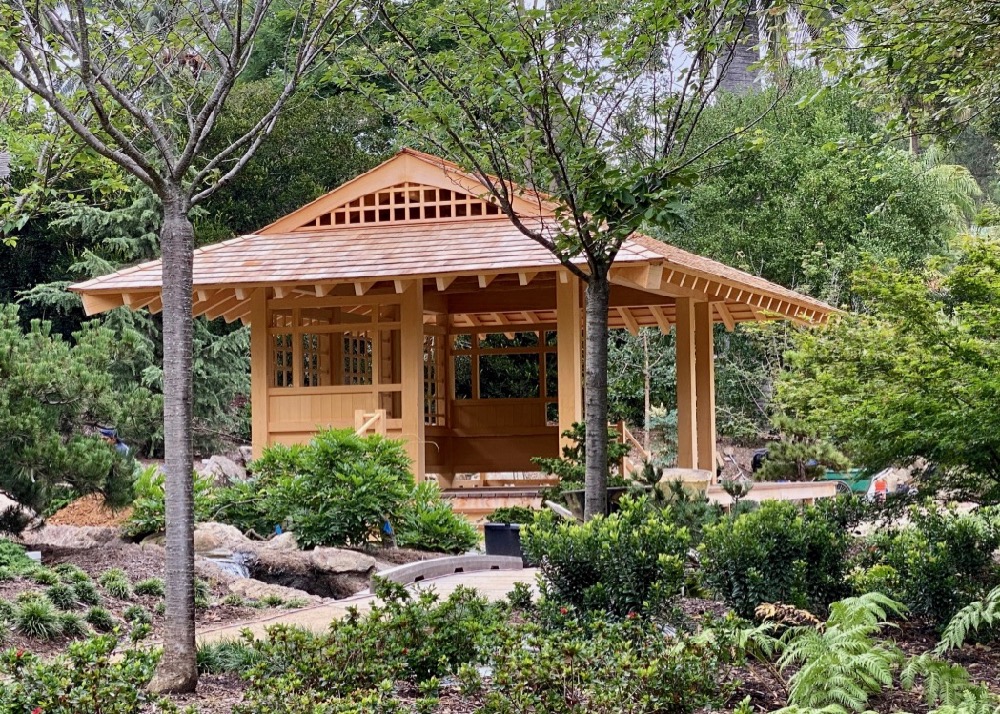The photograph captures a serene outdoor pavilion situated in the heart of a lush garden, bathed in broad daylight. The wooden structure, featuring a bright, blonde hue, evokes an East Asian architectural style with its distinctively inclined roof and intricately arranged beams. The pavilion serves as a semi-open space, ideal for dining or relaxing amidst nature, with some sections walled in while others remain open. Surrounding the pavilion is a thriving array of greenery, including vibrant plants, ferns, shrubs, and tall, healthy trees, all contributing to a verdant landscape. A paved pathway meanders through the garden, leading to the pavilion, and hints at a small bridge, suggesting the presence of a stream nearby. The overall ambiance is tranquil and inviting, enhanced by the clean lines and natural beauty of the setting.